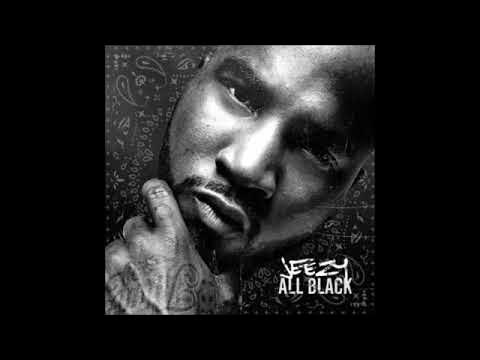The album cover is a square-shaped image set against a black background, featuring a black male artist named Jeezy. Centered within the album cover is a black-and-white photograph of Jeezy, angled diagonally from the top right corner to the bottom left corner. Jeezy's head is slightly tilted to the side, showcasing a serious expression with his hand thoughtfully placed on his chin. His face prominently displays a short black mustache and a neatly trimmed beard, complemented by a shaved head. His hand, which rests near his chin, shows visible tattoos. Jeezy's facial features include a wide nose and full lips. The background of the photograph includes a bandana-like design filled with various shapes. The album's title, "All Black," and the artist's name, "Jeezy," are written in white text located in the bottom right corner of the cover. The emphasis on his facial features and hand, combined with the intricate background and minimalist text, creates a striking and evocative image.